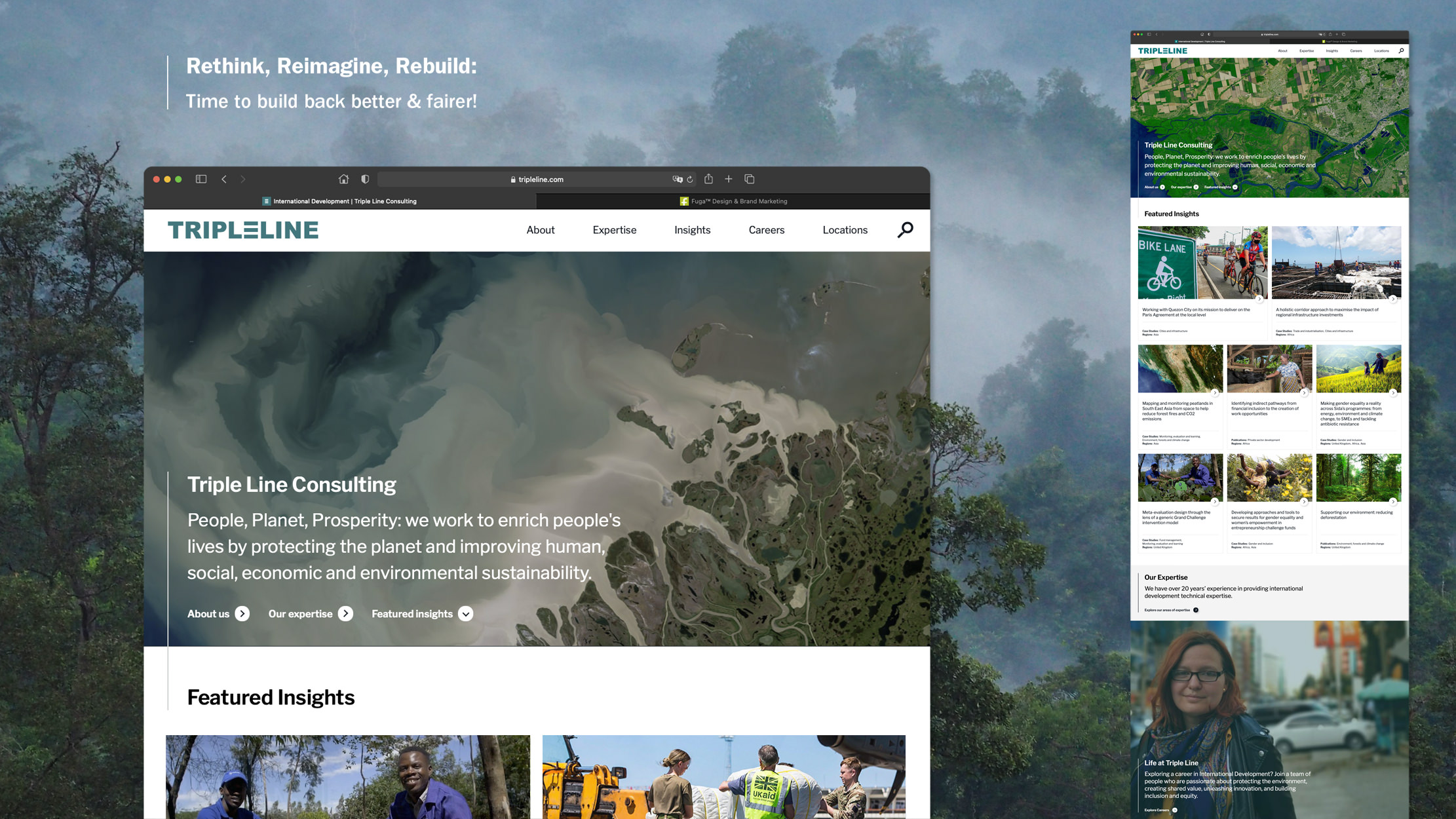This image depicts a web page dedicated to the mission and vision of an organization committed to fostering a more sustainable and equitable world. The text on the page emphasizes the collective effort to "Think, Imagine, Build," underlining a call to action for rebuilding society in a better and fairer way. The organization aims to enrich lives by protecting the planet and enhancing human, social, economic, and environmental sustainability through their specialized expertise in these areas.